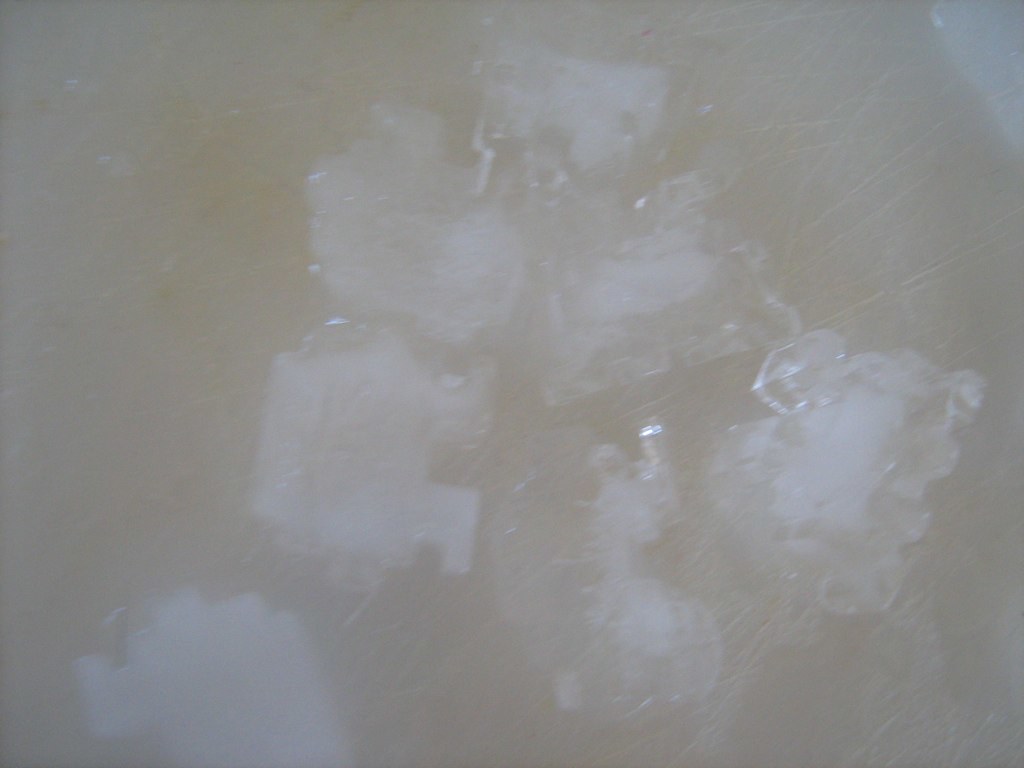The image is a blurry, low-resolution, colored photograph with a soft, yellowish-grayish, or light beige-brown background. In the center, there are a series of indistinct, ice cube-shaped objects that exhibit a hazy, white coloration toward their interiors, fading to clearer edges. These six to seven irregularly shaped objects, resembling jigsaw puzzle pieces more than uniform cubes, are clustered together, possibly melting and resting on a surface that hints at a dimly lit, reflective quality. There is some gentle highlighting on these objects, suggesting light coming from above. However, the overall low quality and out-of-focus nature of the photograph make it difficult to accurately identify the specific details or context of the scene.